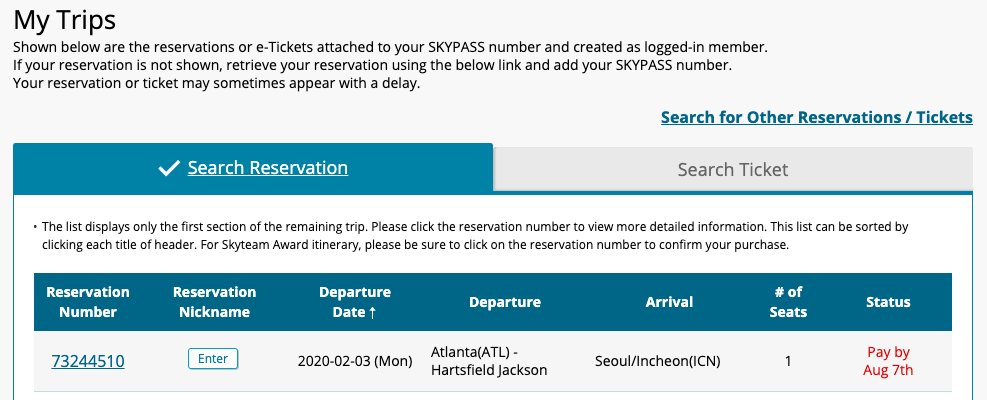This is an image of a "MyTrips" page from a travel management portal. At the top, it displays the "MyTrips" heading, indicating the section of the website where users can view their travel reservations and e-tickets linked to their SkyPass number. The page is designed for logged-in members of the Delta SkyPass program.

The main content of the page shows a list of the user's reservations. If a reservation is not displayed, there is a hyperlink provided to "Search for other reservations and tickets," allowing users to retrieve and add their SkyPass number to any missing reservations. This ensures all reservations are visible, although there might be a delay in appearing.

There are two tabs at the top: "Search Reservation" and "Search Ticket," with "Search Reservation" currently highlighted. This tab informs users that the list displayed includes only the first section of their remaining trips. To view more detailed information, users must click on the reservation number. Users can sort the displayed list by clicking on each column header.

Special instructions are given for Sky Team Award itineraries, advising users to click on the reservation number to confirm their purchase.

Below, there is detailed trip information:
- **Reservation Number:** 732-44510
- **Reservation Nickname:** (Blank for user input)
- **Departure Date:** Monday, February 3rd, 2020
- **Departure:** Atlanta-Hartsfield-Jackson
- **Arrival:** Seoul Incheon International Airport (ICN)
- **Number of Seats:** 1
- **Ticket Status:** To pay by August 7th

The user ends the session with a cheerful sign-off, "Cheers!"